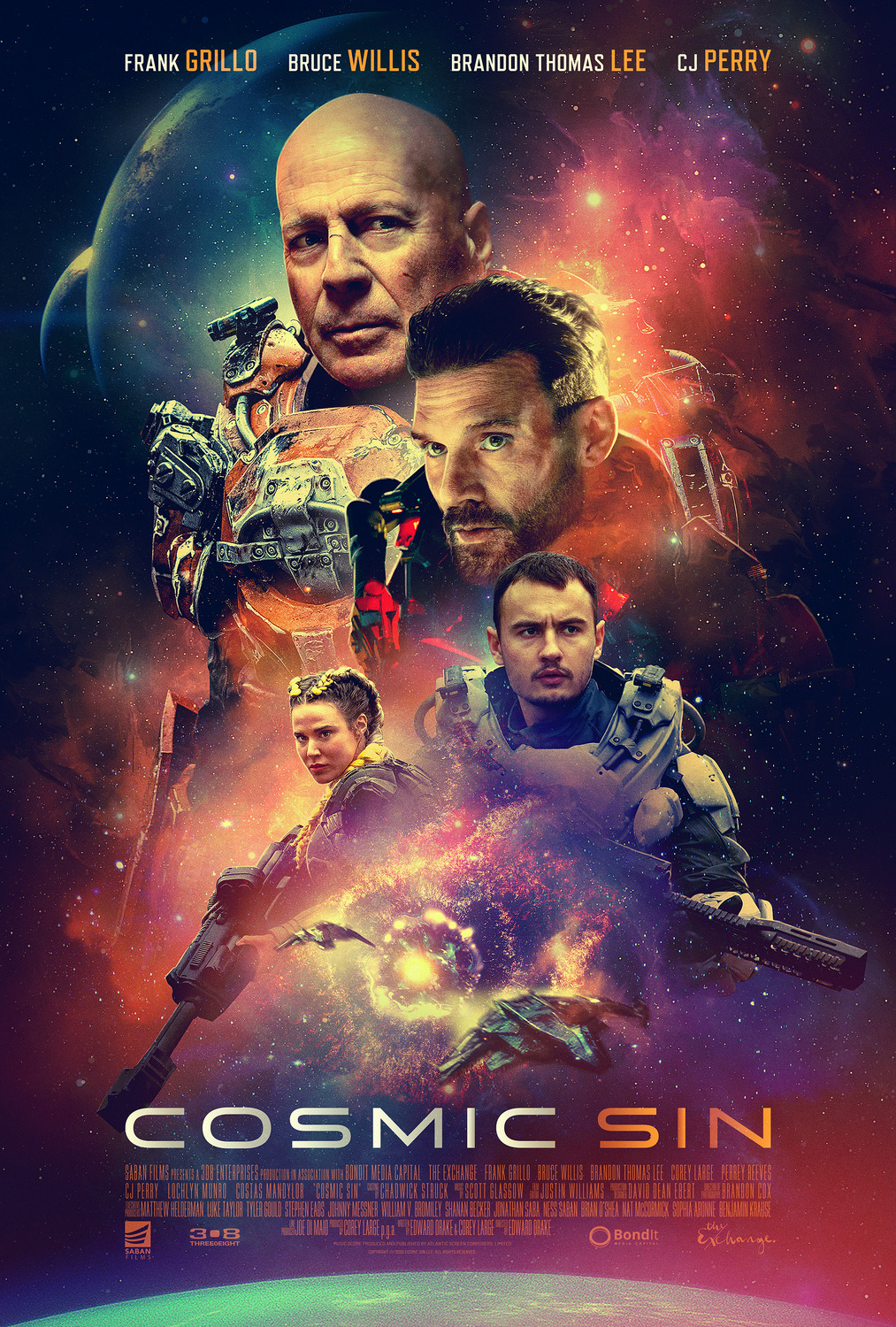This movie poster showcases the film "Cosmic Sin". At the top, the names of the starring actors are prominently displayed. Below the names, the central focus of the poster features an array of characters from the movie, posed in dynamic battle stances or striking tough, contemplative looks, with one character standing prominently at the forefront, making direct eye contact with the viewer. The backdrop suggests a setting in deep outer space, illustrated by two large planets and a multitude of stars scattered across a predominantly black canvas. Adding to the intensity, the scene is punctuated with glaring, red lights that might emanate from battle sequences or bright, glowing stars. The visual elements also include several spaceships and an arsenal of weapons, imbuing the poster with an overall dark and intense atmosphere, contrasted by flashes of bright red. Below the dominant title "Cosmic Sin," additional movie details, including production credits, are neatly listed.